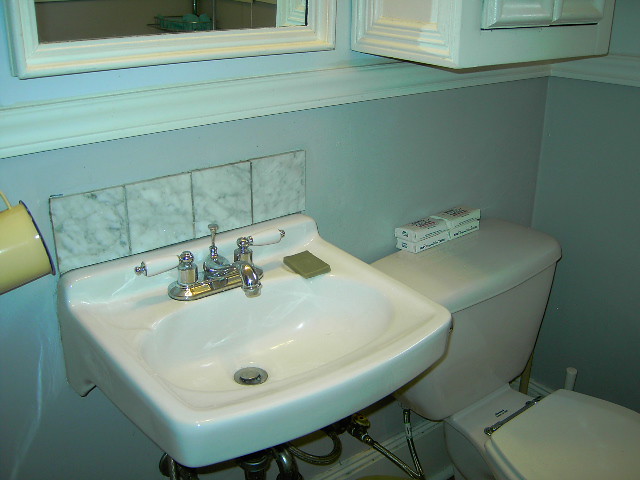The photograph captures the interior of a bathroom. Dominating the lower left quadrant is a white ceramic sink equipped with a chrome faucet. The sink is mounted against a light blue wall, which features a stylish wainscoting rail molding around its midsection. The wall above the molding is a slightly paler, less gray blue, contributing to the room's calming atmosphere. 

Adjacent to the sink, positioned in the lower right quadrant, is a closed-lid toilet nestled in the corner. Above the toilet, a wall-mounted, white cabinet with two doors offers additional storage; it is humorously described as a "real head banger" due to its placement. Resting on the back of the toilet tank are four rectangular packages that are likely to contain feminine hygiene products. A plunger with a white plastic handle is discreetly tucked behind the toilet bowl.

Above the sink, a mirror with a white wooden frame reflects the bathroom's serene decor. The sink area is completed with a four-tile splash guard, also white, adding both functionality and a crisp visual element to the space.